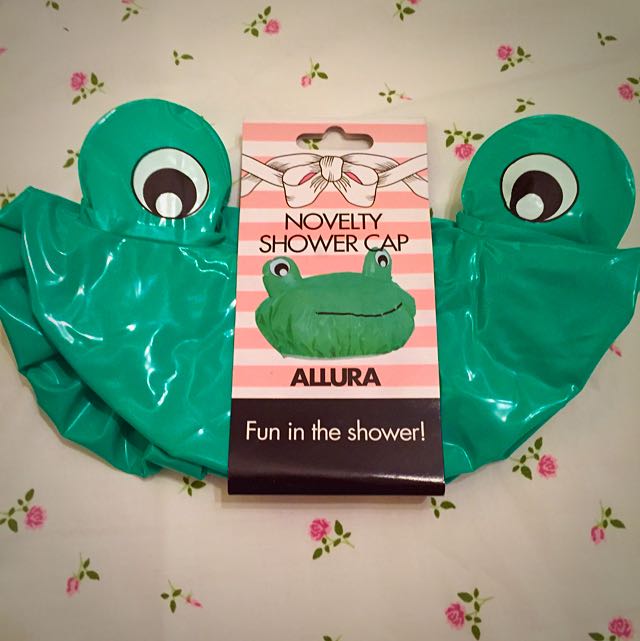This image showcases a novelty shower cap designed to resemble a frog, prominently displayed against a floral background. The shower cap is unopened and is held together by its original packaging, which features a white ribbon design with black lines, and the text "novelty shower cap" written below a whimsical illustration of a frog’s head. The label is a standout with its pink and white striped pattern. The frog motif includes protruding eyes that are detailed with white and black circles, enhancing the playful design. The cap itself is made from green plastic that shines under the light. The branding includes the name "Allura" and the phrase "fun in the shower," indicating a product aimed at adding a touch of humor and enjoyment to a daily routine. The floral background, detailed with purple and pink flowers and green leaves, adds a charming, vintage touch, creating a visually appealing and cheerful composition.